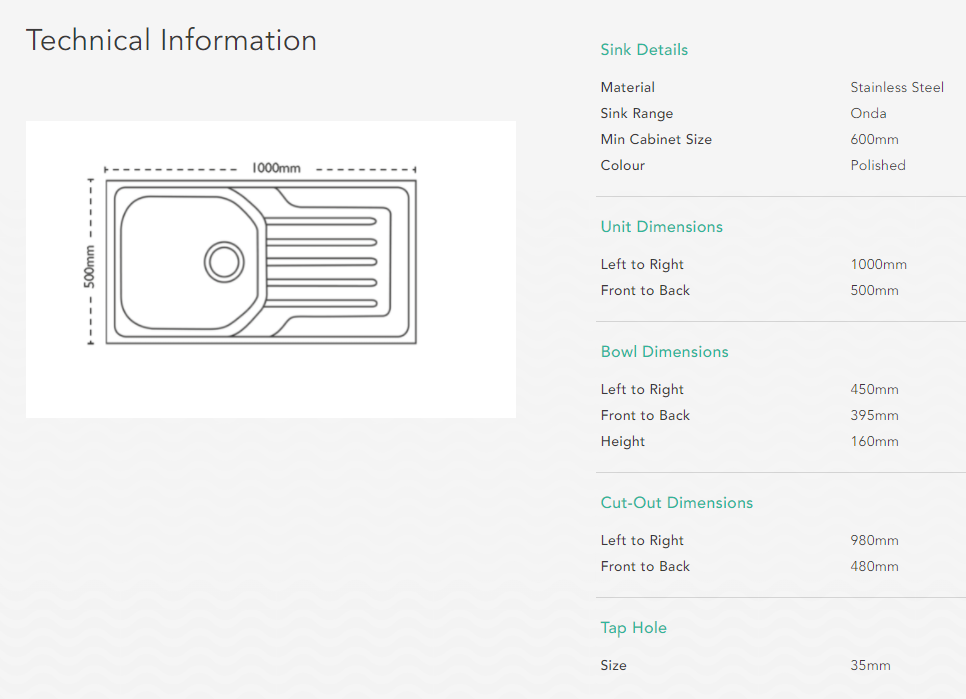**Caption:**

A detailed technical diagram of a stainless steel sink is displayed on a computer screen. The top section is marked by a faint gray square labeled "Technical Information." Below this label, there is a white rectangle featuring a schematic of the sink. This schematic includes dimensions such as "500 mm" (millimeters) running from top to bottom and "1,000 mm" running horizontally. The image also highlights riveted details and a central circle.

Adjacent to the image, organized in green text, is a section titled "Sink Details." Listed information includes the material, defined as stainless steel, and the sink range, noted as Onida or Onda. Minimum cabinet size is specified as 60 mm, and the color is mentioned as polished.

Further down, the unit's dimensions are given as:
- **Left to Right:** 100 mm
- **Front to Back:** 500 mm

Bowl dimensions are also detailed:
- **Left to Right:** 450 mm
- **Front to Back:** 395 mm
- **Height:** 160 mm

Towards the bottom, additional specifications such as cutout dimensions and the tap hole placement are included.